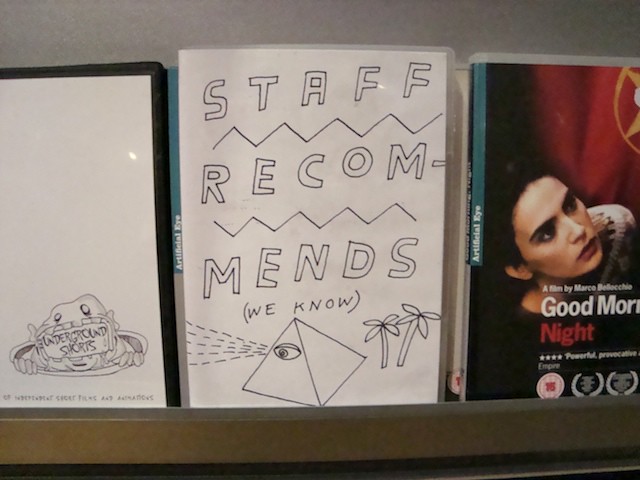The photograph showcases a bookstore shelf displaying staff recommendations. The setting is well-lit, and the objects of interest are positioned vertically. On the left, there is a caricature drawing that features a pyramid with the Eye of Providence, evoking a conspiracy theorist theme. This eye, often seen on the U.S. dollar bill, is set against a backdrop of palm trees and mountains. In the center, a white paper sign with a hand-written note reads, "Staff recommends," with "recommends" split into two lines, connected by a hyphen. Moving to the right, there is a dark-colored DVD case with a red tint titled "Good Morning, Night," a film by Marco Bellocchio. The cover shows a woman, and part of the title is clipped by the edge of the image. The shelving unit itself is brown, adding a warm tone to the bookstore's ambiance. This detailed and eclectic arrangement emphasizes the bookstore's curated selection, appealing to diverse tastes from conspiracy theories to cinematic art.